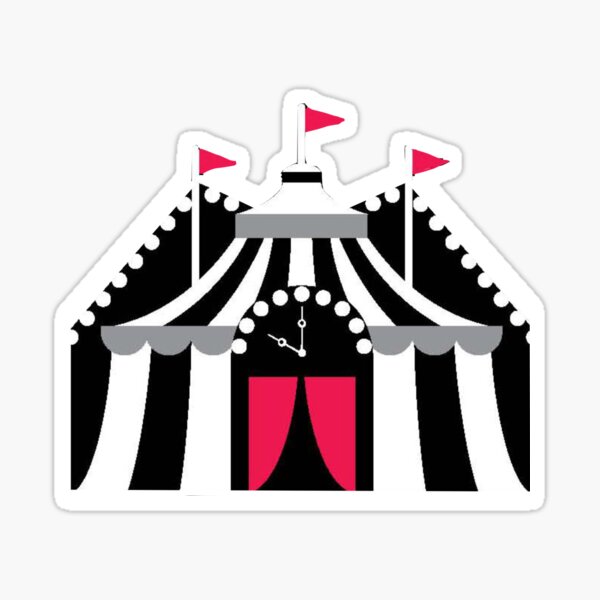This sticker-like illustration showcases a detailed black and white striped circus tent against a light background. The roof of the tent features three tall poles, each topped with a vibrant red triangular flag. The tent’s entrance is emphasized by striking red and black curtains, beneath a semi-circular clock face set to 10 p.m. The top edges of the tent are adorned with small, circular shapes resembling lights. The design captures the festive ambiance of a classic carnival, structured with white poles and accented by subtle gray highlights on the roof’s flaps.